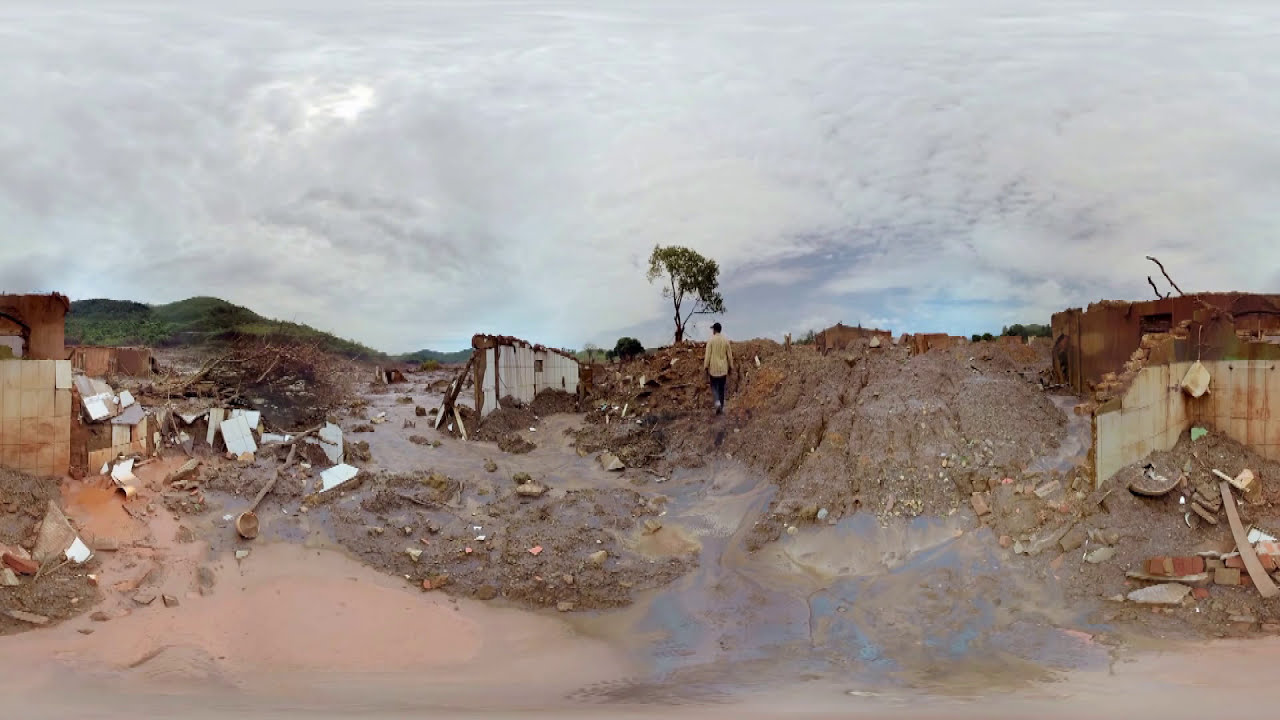The image depicts the aftermath of a devastating event, likely a war or natural disaster, impacting what appears to have been a village. The area is strewn with rubble that includes bricks, stones, and fragments of wood, all remnants of once-standing structures. There are tan and brown remains of buildings, and among the wreckage is a partially destroyed white wall with brown accents.

A person, clad in a light-colored long sleeve shirt, blue jeans, and a black hat, walks through the debris. The ground is covered in rust and brown-colored dirt, interspersed with white and gray rubble and some red bricks. In one area, there is water that looks muddy and bluish, adding to the chaotic and dirty landscape.

Amid the devastation stands a lone tree with some green leaves and brown stems, slightly tilted to the right. In the background, green, lush hills and mountains are visible beneath a sky filled with thick, white clouds. A small sliver of light peeks through these clouds, casting a faint glow over the scene.